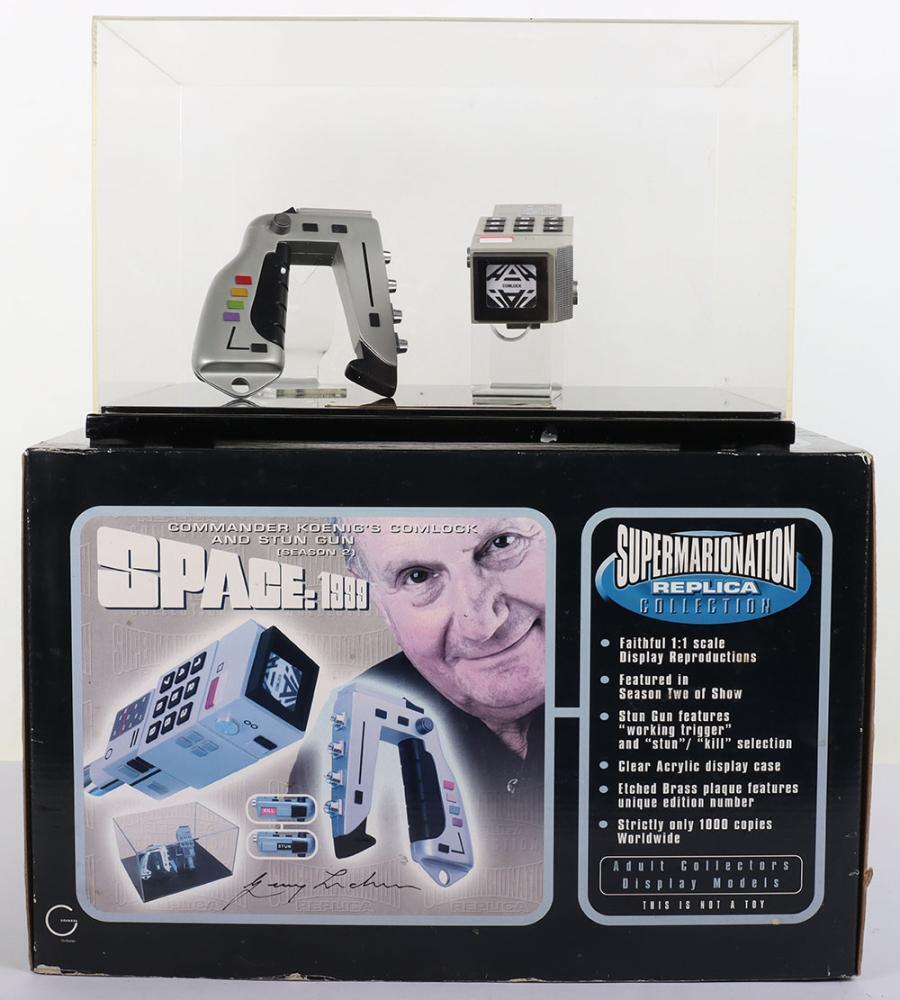The image showcases the cover of a collector's edition device, prominently titled "Commander Koenig's Comlock and Stun Gun," from the vintage sci-fi series *Space: 1999*. This item is part of the Super Marionation Replica Collection and is a faithful one-to-one scale reproduction of the original props featured in the show’s second season. Encased in a clear acrylic display case, the device and its accompanying rectangular module are a drill gray, reminiscent of a futuristic handheld controller, with colorful buttons in red, yellow, green, and purple, as well as numbered buttons and four stainless steel nozzles. The packaging also displays an image of Commander Koenig, portrayed by an older white man, smiling. The black box features various images of the stun gun and detailed breakdowns of its individual components. Notably, the stun gun includes a working trigger with a stun and kill selection switch, and the set comes with an extra brass plaque indicating a unique edition number, emphasizing its rarity with strictly only 1,000 copies available worldwide.